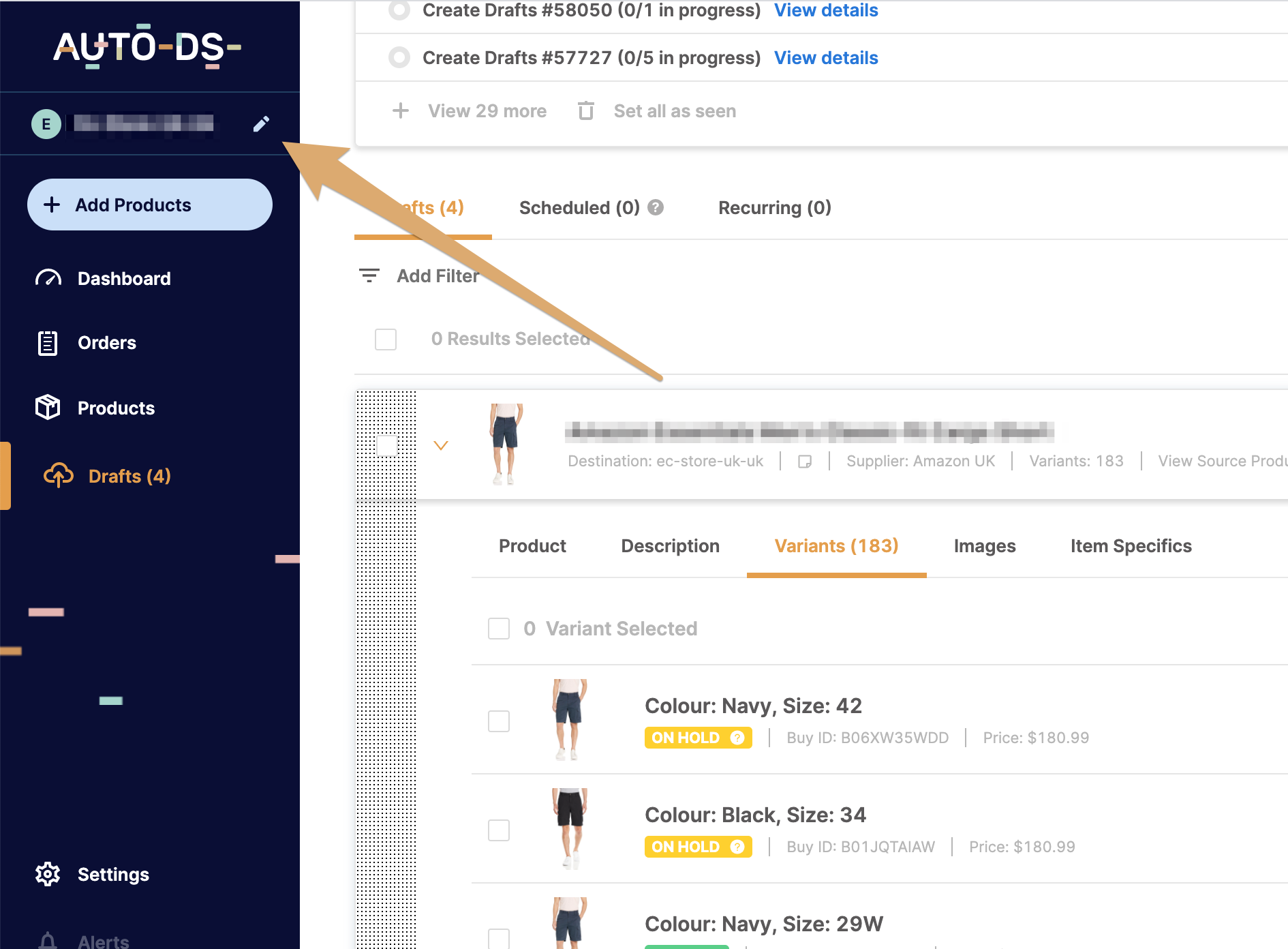This is a screenshot from the Auto DS shopping page. The far left side of the image features a vertical, dark blue rectangle running from top to bottom. The right and middle sections of the image have a white background. At the top left, the Auto DS emblem is displayed. Beneath the emblem, from left to right, there is a light blue circle with a dark blue "E" in the center, followed by a blurred-out name with a tan arrow pointing to it from the right. Below that, there is a light blue oval containing black text that reads "Add Products." Further down, white text lists the following items: "Dashboard," "Orders," and "Products." Below this list, in orange text, it says "Drafts (4)." At the bottom of the menu, "Settings" and "Alerts" are displayed.

To the right of this vertical menu, in black text, it reads "Create Drafts (58,050), 0 of 1 in progress," with a blue "View Details" link next to it. Below, another entry reads "Create Drafts (57,727), 0 of 5 in progress," also with a blue "View Details" link to the right. Underneath, in lighter gray text, it says "View 29 More" and "Set All as Seen."

Further down, there are tabs labeled "Drafts," "Scheduled," and "Recurring," followed by "Add Filter" and "0 Results Selected." Below this, there is an image showing the lower torso and legs of a Caucasian male wearing black shorts and a white top. This section lists: "Destination: EC Store UK," "Supplier: Amazon UK," and "Variants: 183," with a "View Source Product" link beneath.

At the bottom of this section, there are tabs for "Product," "Description," "Variants," "Images," and "Item Specifics." Under the "Variants" tab, it lists selected variants as "Color: Navy, Size: 42," "Color: Black, Size: 34," and "Color: Navy, Size: 29 Wide."